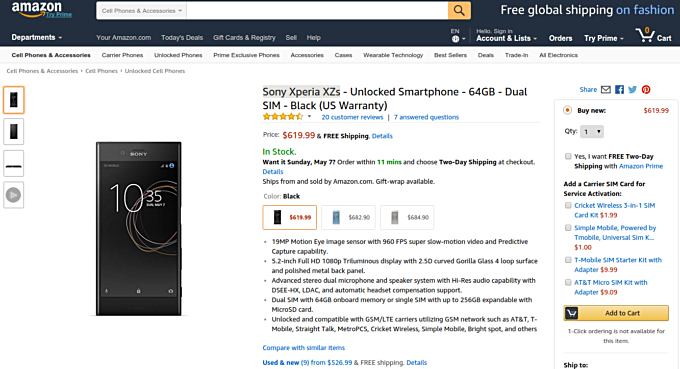This image is a screenshot of an Amazon Prime webpage. At the top left corner, the Amazon Prime logo is displayed. To the right, there is a search bar with an orange search button. Furthermore, the phrase "FREE GLOBAL SHIPPING" appears in white text next to "ON FASHION" in blue text. The entire upper background of the webpage is black.

Beneath the main navigation bar, there are various categories listed: "Departments," "YourAmazon.com," "Today's Deals," "Gift Cards & Registry," "Sell," and "Help." Adjacent to these, on the same line, are sections for "Account & Lists," "Orders," "Try Prime," and a shopping cart icon indicating there are currently zero items in the cart.

Below this navigation menu are 11 smaller categories, with the current focus on "Cell Phones & Accessories." Featured prominently on the page is the Sony Xperia XZS Unlocked Smartphone with 64GB of storage and dual SIM capabilities in black. The price is displayed in red as $619.99. To the left of this price is an image of the phone, accompanied by four smaller images showcasing the phone from different angles, stacked vertically.

The availability status is shown in green text stating "In Stock." The phone color is black, but it appears there are three color options available. There are five lines of small black text detailing different features of the phone. 

To the right, there are options for purchasing: a "Buy Now" button, various clickable links, and an "Add to Cart" button in a yellow rectangle. The bottom half of the page has a white background, contrasting the black top section.